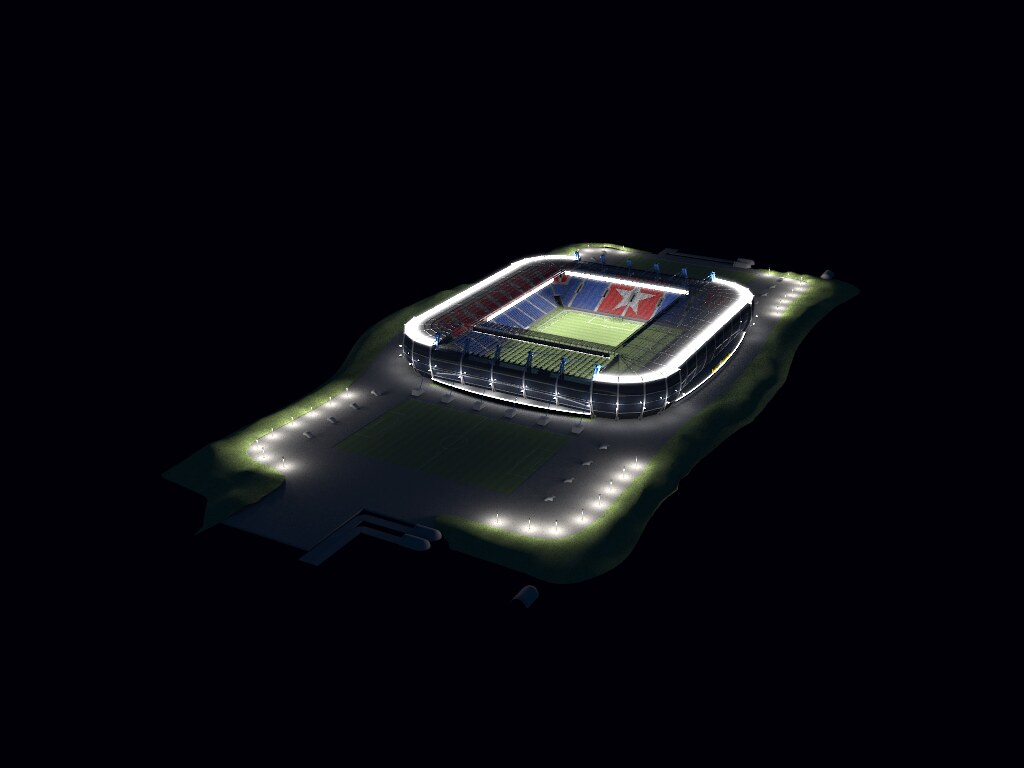A far aerial 3D rendering of a stadium dedicated to an unspecified sport is showcased against a vast black background, making it appear as though it is floating within a black void. The stadium is square with see-through mesh covering the seating areas, which are adorned in vibrant blue, red, and white, forming a star design. Inside, the green playing field features multiple white lines and markings, along with goalposts. Notably, the stadium is surrounded by lit parking lots in both the front and back, though these lots are empty. The edges of the parking lots are illuminated by lights, enhancing the surreal floating effect against the dark backdrop.